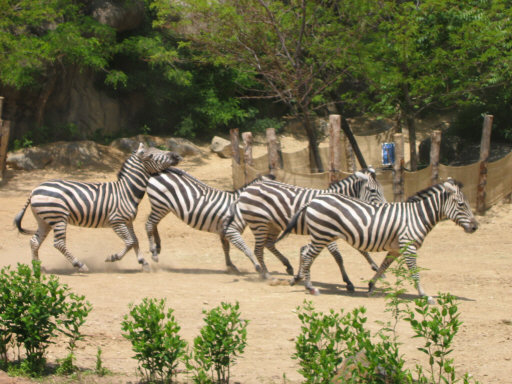A lively photograph captures a line of four zebras walking from left to right against a backdrop of natural scenery. The image, slightly hazy yet colorful, showcases the zebras in various dynamic poses. Each zebra is adorned with striking black and white stripes and the front zebra sports a distinctive mohawk-style mane. The rear zebra endearingly rests its chin on the rump of the zebra ahead, adding charm to the scene. Surrounding the zebras, the ground is a sandy, almost hard surface, dotted with small green bushes and rocks. In the background, towering trees with brown trunks and green leaves are encircled by protective barriers, likely to prevent animals from getting too close. A fence made of fabric and wooden pillars is also visible, hinting at a location such as a zoo. The photograph is devoid of text, focusing purely on the beauty and camaraderie of the zebras amidst their serene environment.